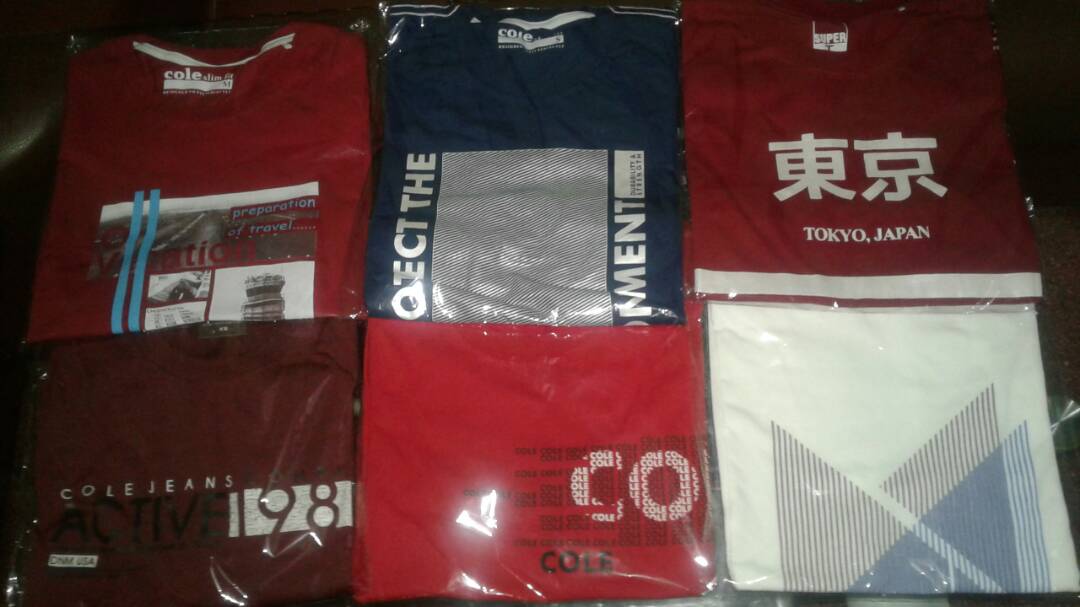The photograph captures a collection of six t-shirts wrapped in plastic packaging, seemingly prepared for sale or display in a store. The shirts are arranged in two rows, each with distinct colors and logos. In the top row, the first t-shirt is a bright red one featuring the brand "Cole" on the upper front. Next to it is a black and white t-shirt, also branded "Cole," though its exact design is obscured due to folding. The middle shirt in this row is another red t-shirt, showcasing "Tokyo, Japan" in white block letters with two Han characters above. 

In the bottom row, the first shirt is maroon and reads "Cole Jeans Active 98" across the front. The fifth item is a vibrant red t-shirt partly visible, showing "CO" with the rest of the design folded, and the word "Cole" in black lettering below. The last shirt in the collection is white, displaying an indeterminate black and white design due to its partial folding.

The photograph is slightly blurry and appears to have been taken in a dimly lit room, contributing to the overall impression that these t-shirts are either being prepped for retail or already set for a store display.